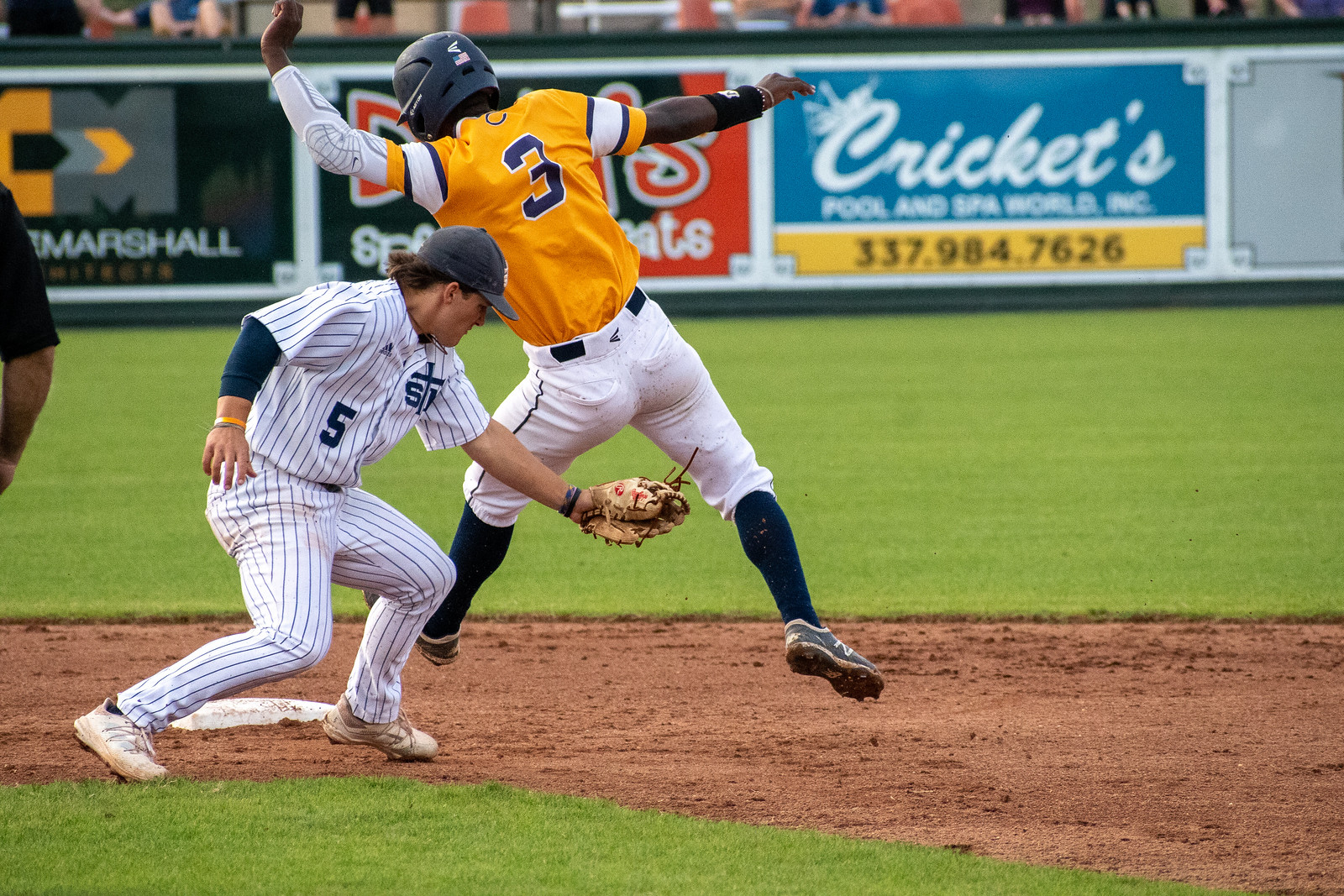This is a horizontal rectangular image capturing an intense action scene from a baseball game. In the center of the photograph, a player in an orange jersey and white pants, wearing a black helmet and black socks, is racing toward a base. The runner's arm is clad in a protective wrap, while the other arm remains bare. His opponent, dressed in a white pinstriped uniform with the number five and a black cap, is leaning in with a glove attempting to tag him. The pinstripe player's shoes are white. The base is visible on the left-hand side, surrounded by a brown dirt track that contrasts with the green grass of the baseball field. In the background, there is a wall adorned with various advertisements, marking the beginning of the spectators' stands. The ads include mentions of "Marshall" and "some kind of meat" on the left, and "crickets, pool and spa" with a phone number on the right. The photograph captures the moment of suspense and athleticism in vivid detail.